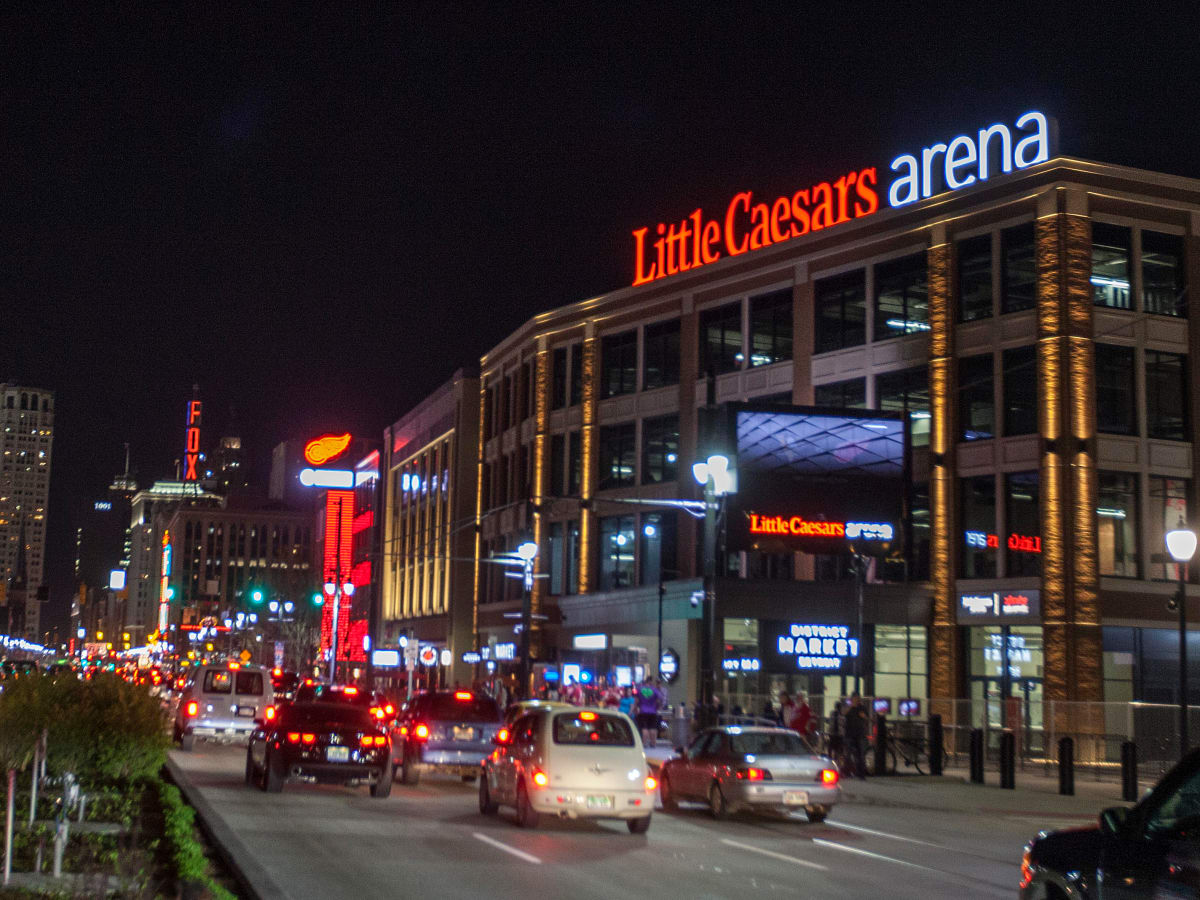The nighttime cityscape captures a bustling downtown area dominated by the well-lit Little Caesars Arena. The dark sky is devoid of stars or planes, creating a contrasting backdrop for the brightly illuminated buildings and streets. Little Caesars Arena stands prominently with its glass windows and multiple levels, supported by gold pillars. Its name shines in vivid neon, with "Little Caesars" in orange and "arena" in white lowercase letters. 

In the foreground, a steady stream of traffic fills a four-lane road, with the glow of red, white, and yellow car lights creating a dynamic scene. To the left of the arena, a high-rise building shows sporadically lit offices or apartments, while lower to the ground, bushes and plants line the curb. 

To the right, another well-lit building features unreadable neon signage bordered by yellow flames trimmed in red lights. In the background, the iconic Fox Theater sign stands out in large red neon letters. The streets are alive with movement as vehicles navigate the city, turning left down the road in front of the arena and adding to the vibrant nocturnal energy of the scene.